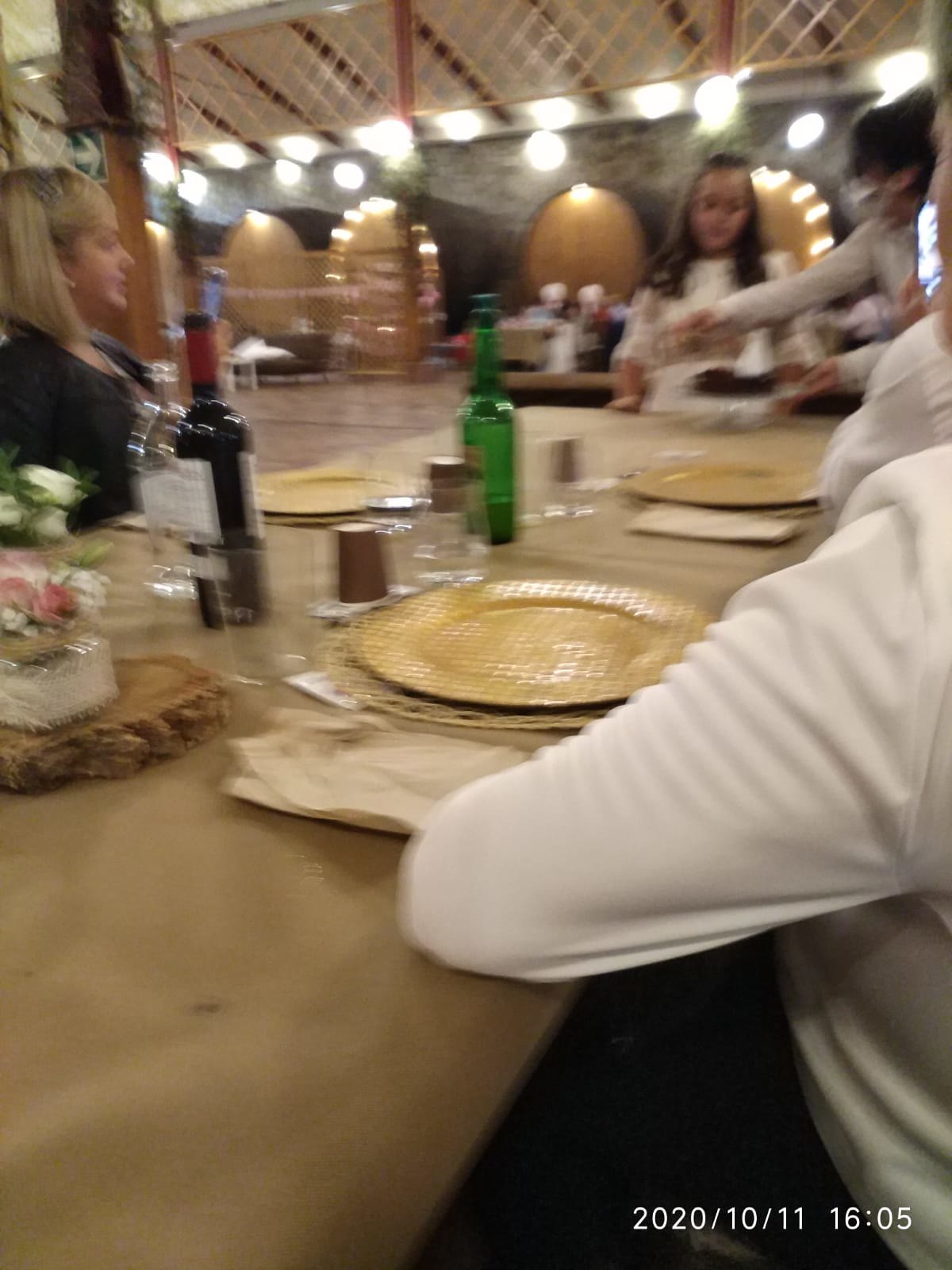This slightly blurry image, likely taken by a phone or security camera, captures a family dinner setting on October 11, 2020, at 16:05, as indicated by the timestamp at the bottom right. The scene unfolds around a long brown table adorned with a tan tablecloth and gold plates, each accompanied by off-white napkins placed on the left. Central to the table's decor is a floral centerpiece resting on a circular mat with a cut tree stump beneath it, housing white and pink flowers in a white pot. Multiple bottles are visible, including a red wine bottle with a white label and a green bottle, suggesting possibly white wine.

Seated around the table are four distinguishable individuals: a person in a white long-sleeve top, another in a grayish top with blonde hair, and a person in black. One person on the right is standing, and two people at the head of the table, both dressed in white, can also be seen. The backdrop features gray arches adorned with lights, adding a festive ambiance to the pavilion-like setting. Brown and possibly pepper shakers alongside various wine glasses further enhance the detailed dining arrangement, capturing a cozy and intimate family gathering.